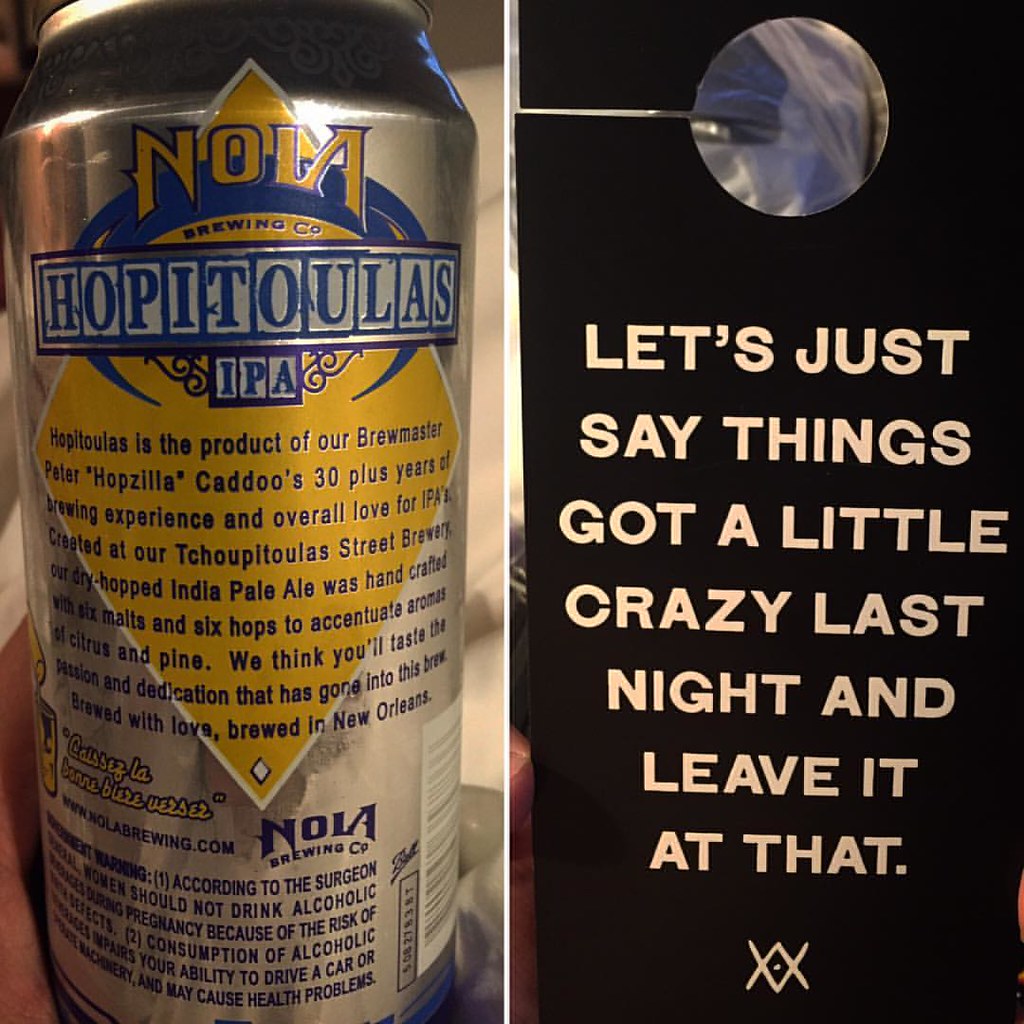This image is vertically split into two sections. On the left half is a silver beer can from NOIA Brewing Company. The can prominently features the label "Hapitolis IPA" inside a yellow diamond-shaped banner, which is filled with additional detailed text about the product. Below the diamond, more text is featured, indicating the product's specifics such as it being crafted by brewmaster Peter Hop with over 30 years of brewing experience, showcasing the quality and heritage of the IPA. The can also mentions safety information and hints that it is brewed in New Orleans.

The right side of the image is a black rectangle with a small circular cutout at the top. In yellowish letters, it reads, "Let's just say things got a little crazy last night and leave it at that XX." This side contrasts with the detailed product information on the left, suggesting a playful and perhaps adventurous narrative associated with the beer.